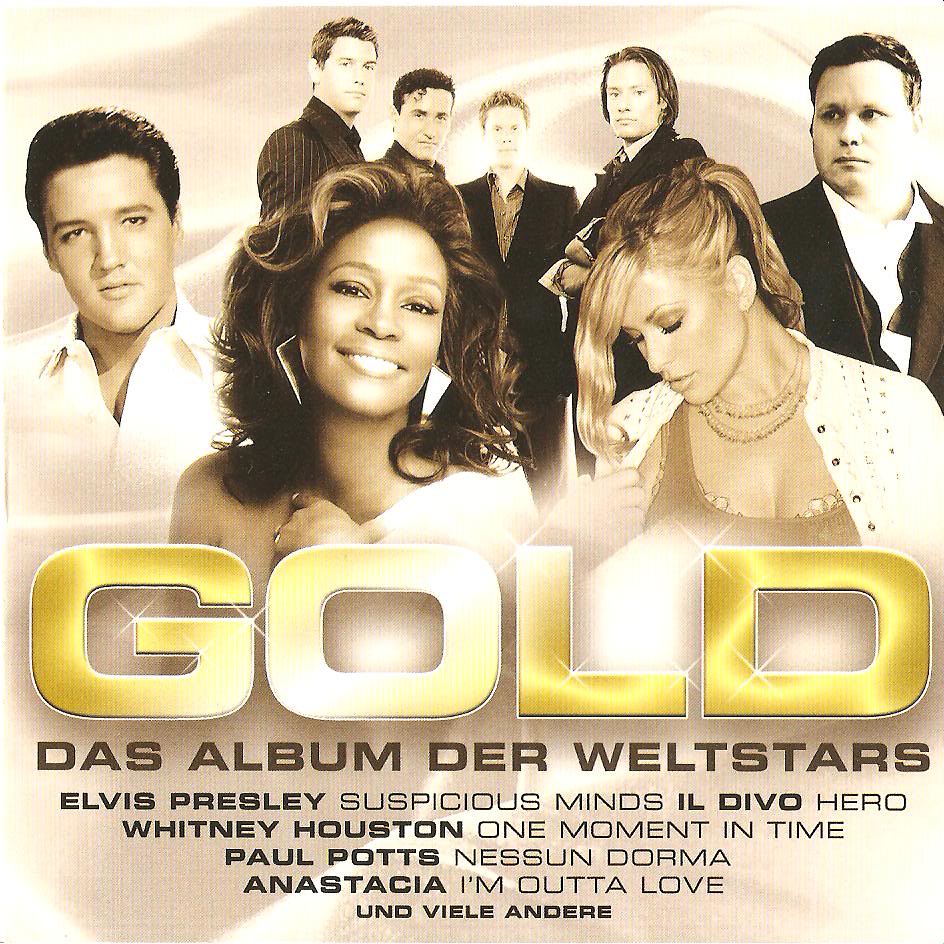The image is an album cover featuring the title "GOLD" prominently displayed in gold letters. Below the title, written in brown or black, is the tagline "Das Album der Weltstars," followed by a list of artists and their famous songs: Elvis Presley with "Suspicious Minds," Il Divo with "Hero," Whitney Houston with "One Moment in Time," Paul Potts with "Nessun Dorma," and Anastasia with "I'm Outta Love." The cover has a sepia-toned background and prominently features multiple iconic artists. In the foreground, Whitney Houston is positioned centrally, flanked on her left by Elvis Presley in a white open collar button-down shirt and on her right by a blonde woman in a tan tank top with a white coat draped over her shoulder. In the back, Paul Potts is featured in a suit next to a group of four men in black suits, who are members of Il Divo. The overall design emphasizes the star power and classic appeal of the artists featured on the album.